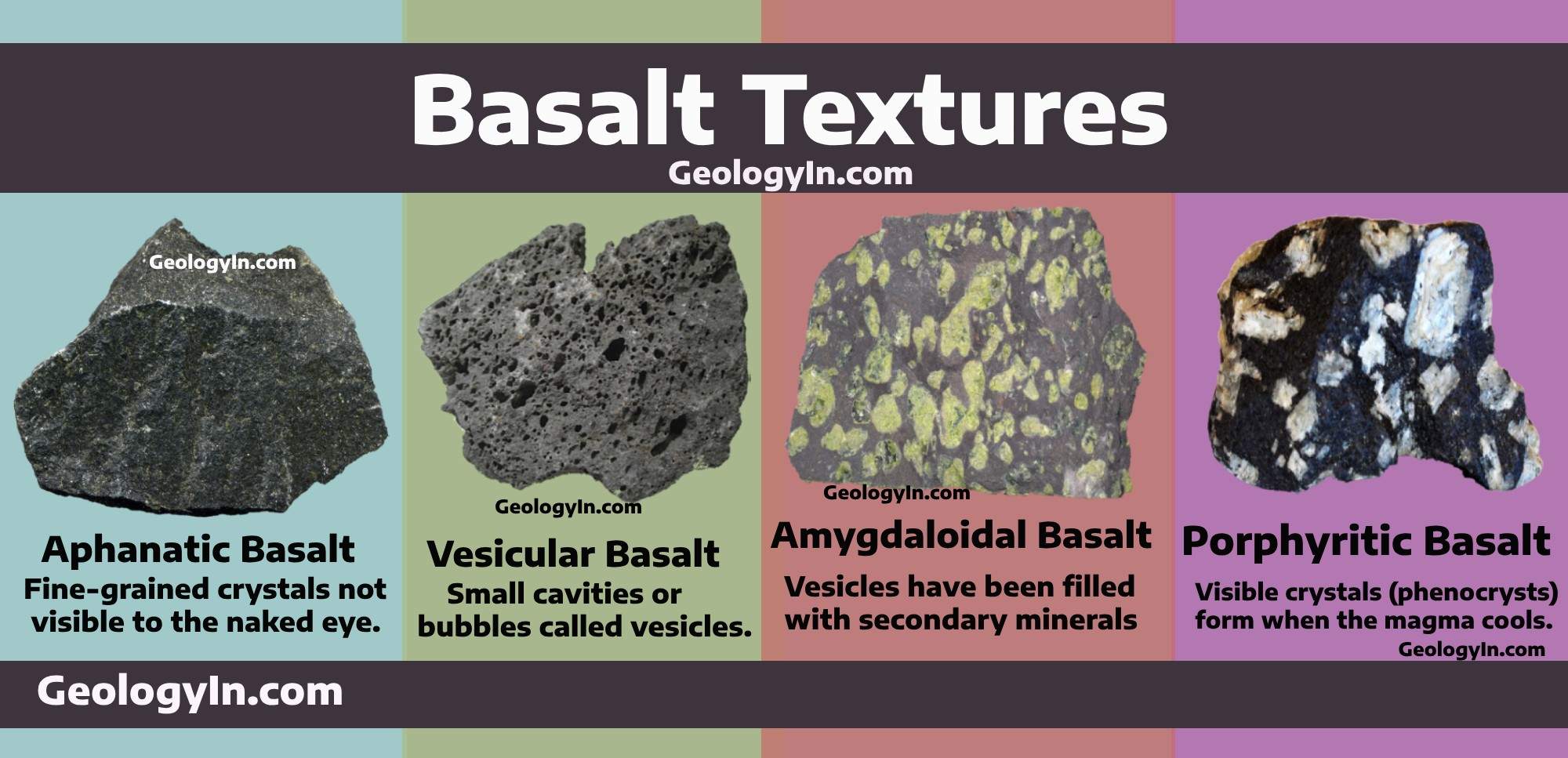The image is an informative graphic on different basalt textures, featuring the title "Basalt Textures" in prominent white letters at the top, followed by the website "geologyin.com." The image is divided into four distinct sections, each highlighting a different type of basalt. 

1. **Aphanitic Basalt:** Set against a blue background, this type is described with "Fine-grained crystals not visible to the naked eye."
2. **Vesicular Basalt:** On a green background, it shows "Small cavities or bubbles called vesicles."
3. **Amygdaloidal Basalt:** Displayed on a reddish background with green dots, it explains that "Vesicles have been filled with secondary minerals."
4. **Porphyritic Basalt:** Featuring a purple background, it details that it has "Visible crystals (phenocrysts) formed when the magma cools."

At the very bottom, the graphic is concluded with "geologyin.com" in a long black stripe.